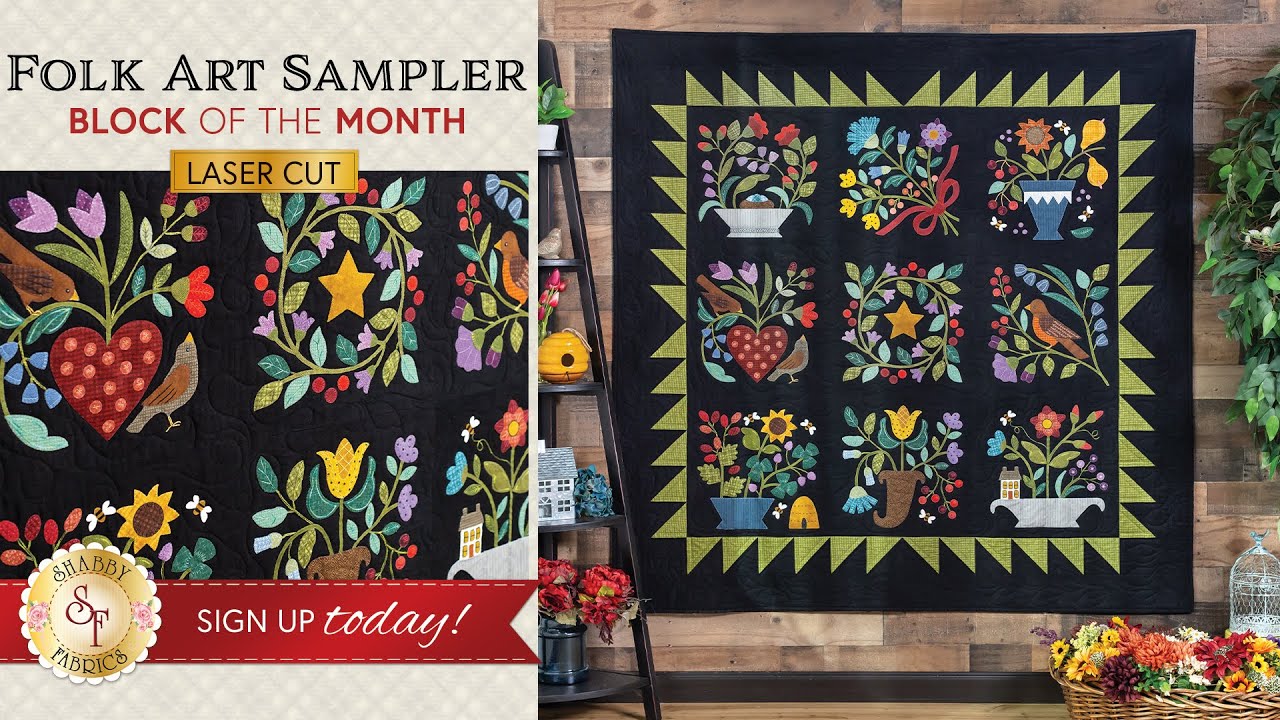The image is a promotional advertisement for the "Folk Art Sampler Block of the Month" laser-cut quilt project by Shabby Fabrics. The photo prominently displays a beautifully quilted blanket hanging on a wall with wooden paneling. The quilt features a striking dark blue background, bordered by a pattern of golden triangles. Within this frame, a 3x3 grid of nine unique and colorful blocks showcases various designs, including flowers, birds, stars, hearts, and potted plants, each with intricate details such as stems, berries, leaves, and garlands. The right side of the image includes a photograph of the completed quilt, illustrating the craftsmanship and vibrant decorations. At the bottom, there's a red banner ribbon encouraging viewers to sign up early, accented by the Shabby Fabrics logo. The scene is set in a cozy store, adorned with baskets of flowers and greenery, enhancing the festive and inviting atmosphere of the advertisement.